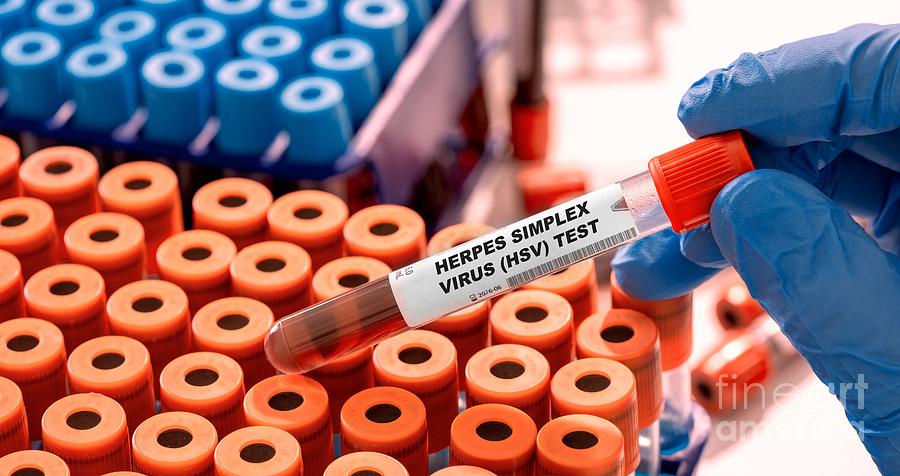The horizontal-rectangular image depicts a detailed laboratory setting. Central to the image is a human hand clad in a dark blue protective glove, holding a test tube with a red cap. The test tube's label reads "Herpes Simplex Virus (HSV) Test" and contains a reddish liquid on one side. On the right side of the image, the gloved hand is prominently featured, emphasizing the significance of the test tube. 

In the foreground to the left and center, there is a well-organized grid of vials with orange tops, arranged in rows. Behind these, in the upper left corner, additional vials with blue tops are visible, creating a contrasting background that helps distinguish the two sets of samples. Near the blue-gloved hand, on the tabletop, more vials can be seen laying flat, adding to the sense of a busy, well-stocked lab. The upper right corner has a white background, further emphasizing the laboratory environment. The image is meticulously composed, highlighting the precise nature of viral testing being undertaken.